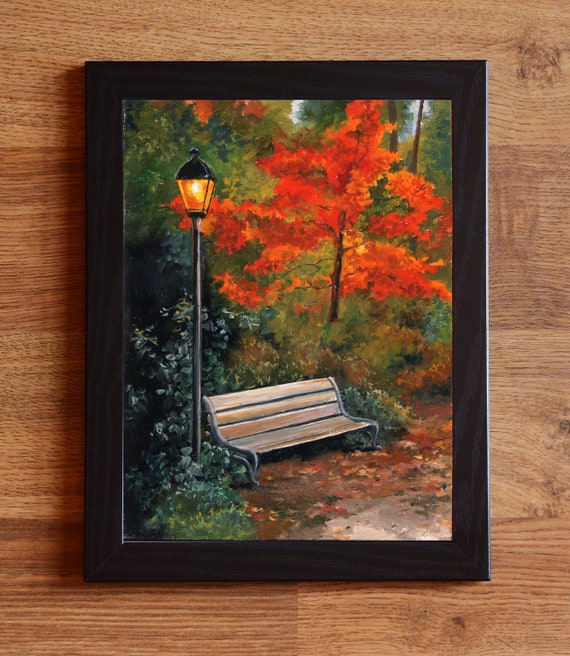This photograph captures a framed oil painting set against a dark brown oak wood floor. The painting, enclosed in a simple black frame, depicts a serene autumn park scene. Central to the image is a wooden park bench, placed prominently as the focal point. To its left stands a classic black street light with a rhombus-shaped glass lantern and a black cap, reminiscent of traditional London lampposts. The light from the lantern emits a warm orange glow. Surrounding the bench are various shades of green bushes, adding depth to the scene. Dominating the background is a majestic tree, possibly a maple, with vibrant, bright orange leaves that suggest the peak of fall. Patches of blue sky can be seen behind the tree, while scattered autumn leaves decorate the ground, enhancing the seasonal ambiance.